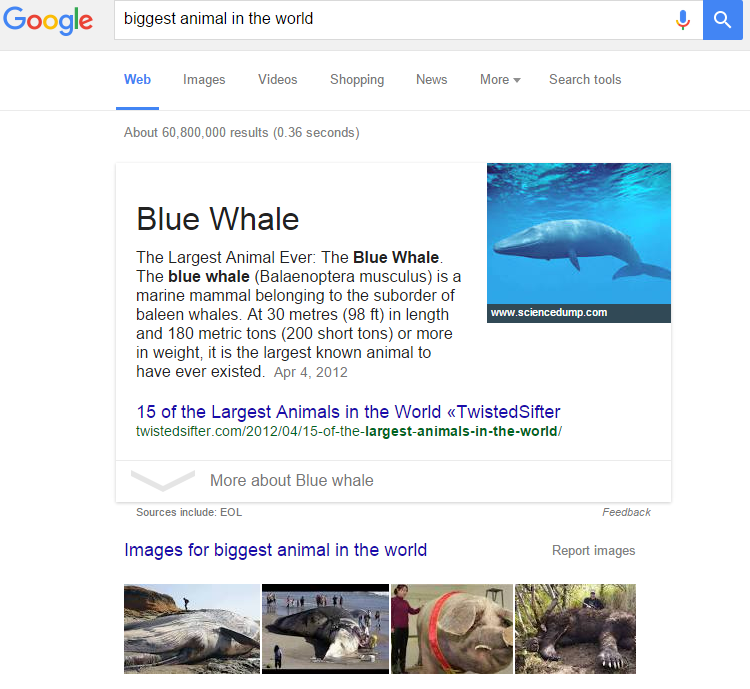Screenshot of a Google Search Page

This image captures a Google search results page with a grey header at the top, prominently featuring the Google logo on the left. In the center of the header is the search bar, which contains the query, "biggest animal in the world" typed in lowercase font. On the right side of the search bar, a microphone icon for voice typing and a search icon are visible. The main body of the webpage is white, creating a clean backdrop.

Centered just below the search bar, Google offers various search options: Web, Images, Video, Shopping, News, More, and Search Tools—with "Web" highlighted. Underneath these options, it's indicated that there are approximately 60,800,000 results, fetched in 36 seconds.

The first search result answers the query, identifying the blue whale as the biggest animal in the world. To the right, there is a thumbnail image of a blue whale, accompanied by the source and website link. On the left, a brief description of the blue whale is provided, along with another link for further reading. Below this section, a drop-down box offers more details about the blue whale.

At the bottom of the webpage, there's a section titled "Images for biggest animal in the world," displaying four thumbnail images related to the search query.